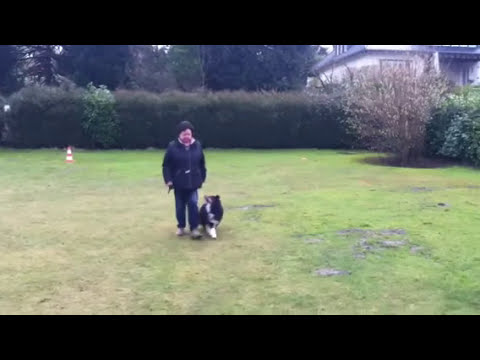The image depicts an outdoor scene featuring a short, light-skinned woman of Asian descent walking her black and white mid-sized dog. She is captured heading towards the camera in a wide rectangular frame cropped with thick black rectangles at the top and bottom. The woman, with her short brown hair, dons a zipped-up black jacket, dark-colored pants, and beige shoes. The dog's gaze is fixed upon her.

The backdrop showcases a bright green lawn with meticulously trimmed short grass, spanning a quarter-acre or less. Encircling the upper part of the image is a dense, dark green shrubbery wall, with towering trees behind it. Towards the right side, among the shrubbery, there’s a tree bearing white flowers, and a mainly white house with gray accents is visible in the top right corner. Additionally, an orange and white cone stands in the field, positioned towards the upper left. The vivid setting, cast in natural daylight, emphasizes a clear and bright day with no other people or animals in sight.